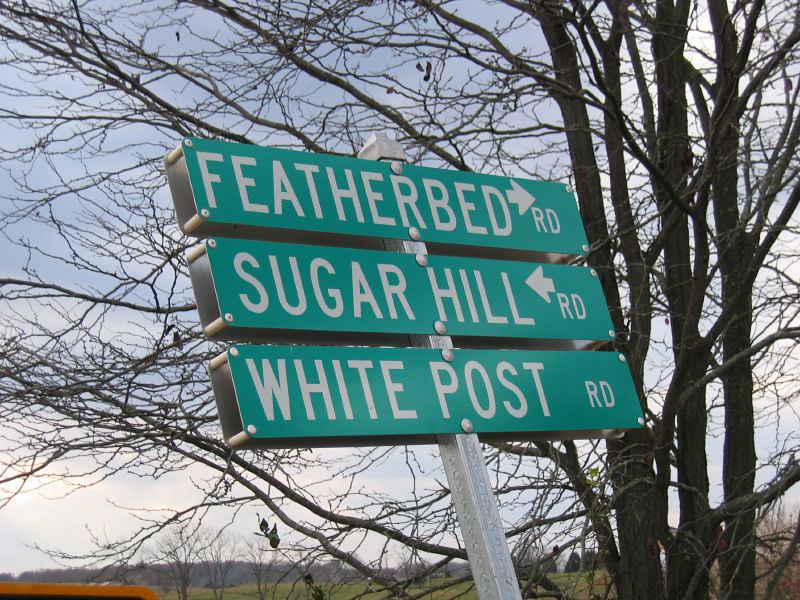In this daytime outdoor photograph, we observe a scene featuring three distinct street signs mounted one above the other on a single silver pole. Each sign is green with white lettering, enhancing their visibility. Starting from the top, the first sign reads "Featherbed Road" and includes an arrow pointing to the right, indicating the direction of the road. Directly below it, the second sign reads "Sugar Hill Road" with an arrow pointing to the left, guiding travelers. The final sign at the bottom reads "White Post Road" without any directional arrow attached. Surrounding the signs, the landscape is adorned with numerous trees, most of which are stark and nearly barren, featuring only a few leaves clinging to their branches. The horizon in the background reveals a blend of low-lying trees and patches of grass, completing the serene, natural backdrop of this image.